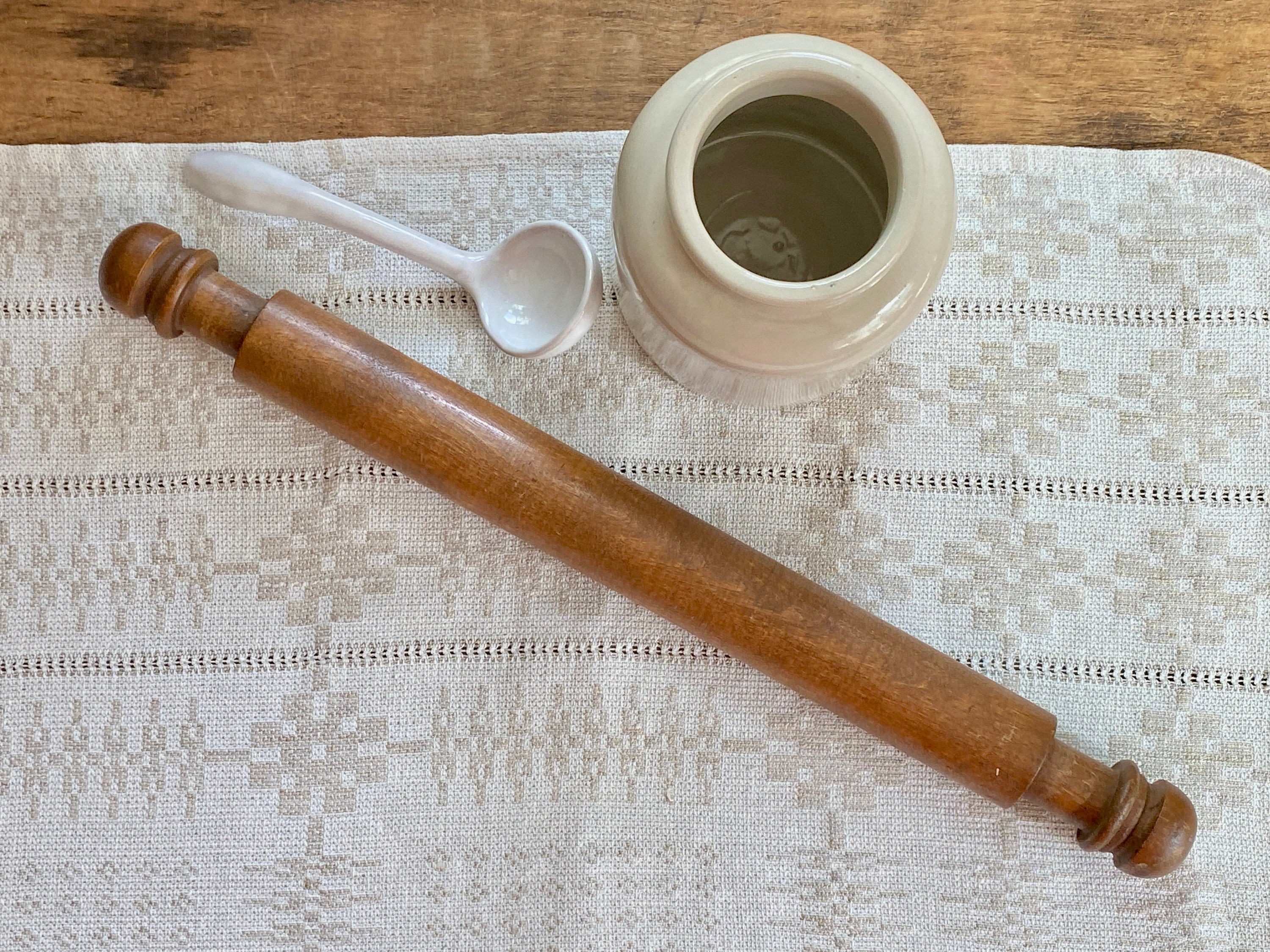The image depicts a scene on a wooden table covered with a cotton tablecloth featuring a white and gray floral pattern. Central to the setup is an antique-style wooden rolling pin, well-worn but meticulously maintained, characterized by its long, smooth rolling surface and hand-carved handles. Adjacent to the rolling pin, positioned to the left, is a small, white ceramic ladle, perfectly sized to fit into the mouth of a nearby ceramic dish. This dish, possibly a caster with a narrow mouth, stands out with its white ceramic construction. Together, these rustic kitchen tools create a nostalgic tableau of traditional baking implements.